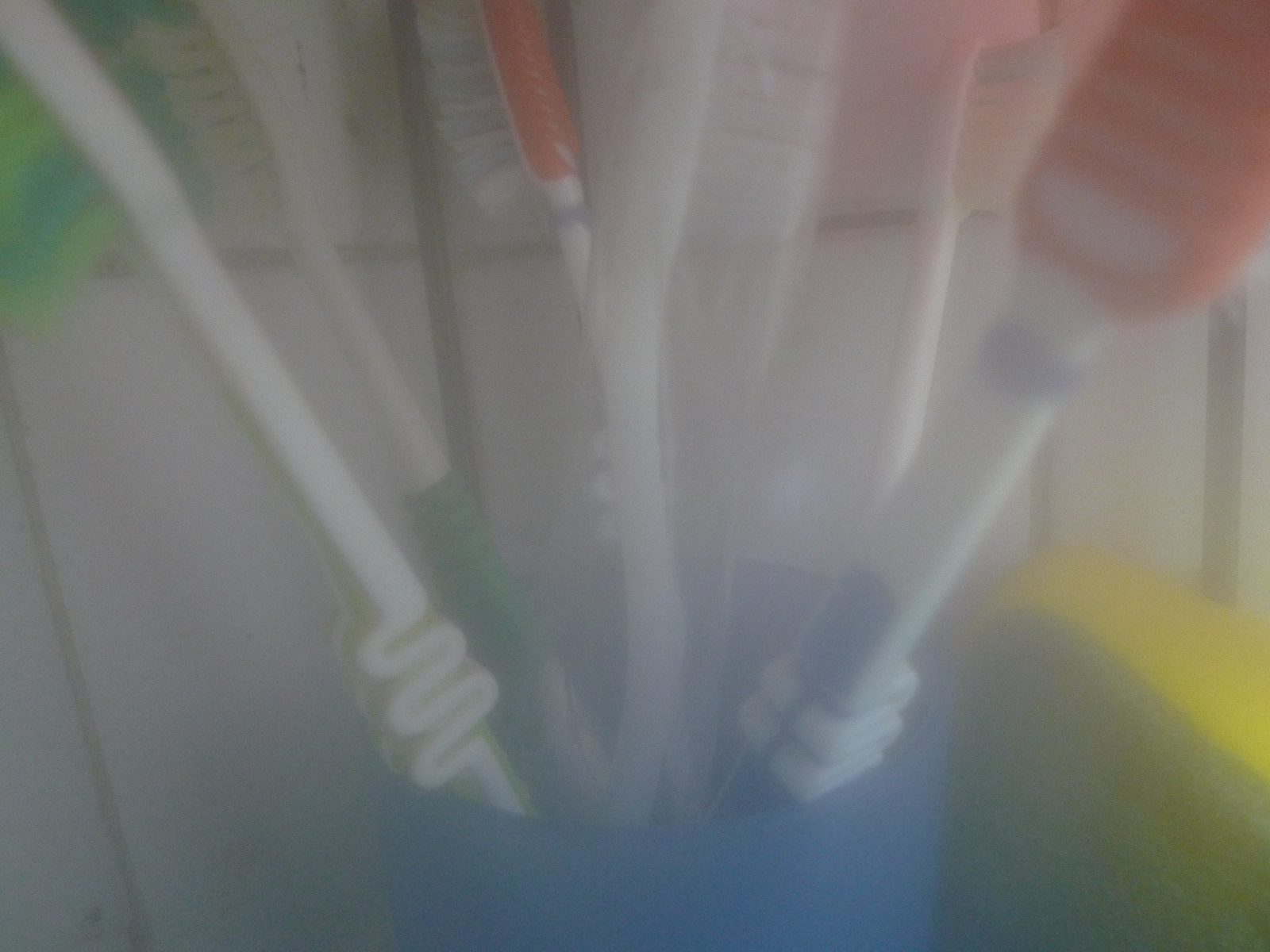This is an extremely blurry and grainy real-life image, possibly taken accidentally, of seven toothbrushes standing in a blue plastic cup. The image is rectangular and displayed in landscape mode, with a very zoomed-in perspective that cuts off the top of the toothbrushes. Each toothbrush has a white handle with a zig-zag pattern for better grip, and the bristles are various colors—green, blue, orange, and white. The background is indistinct, but contextually it appears to be a bathroom setting. To the right of the cup, there is a barely visible yellow and green container, possibly a sponge, further suggesting the domestic bathroom environment. Despite the poor quality, the close-up clearly shows the dense arrangement of the toothbrushes, raising curiosity about the shared use of this space.